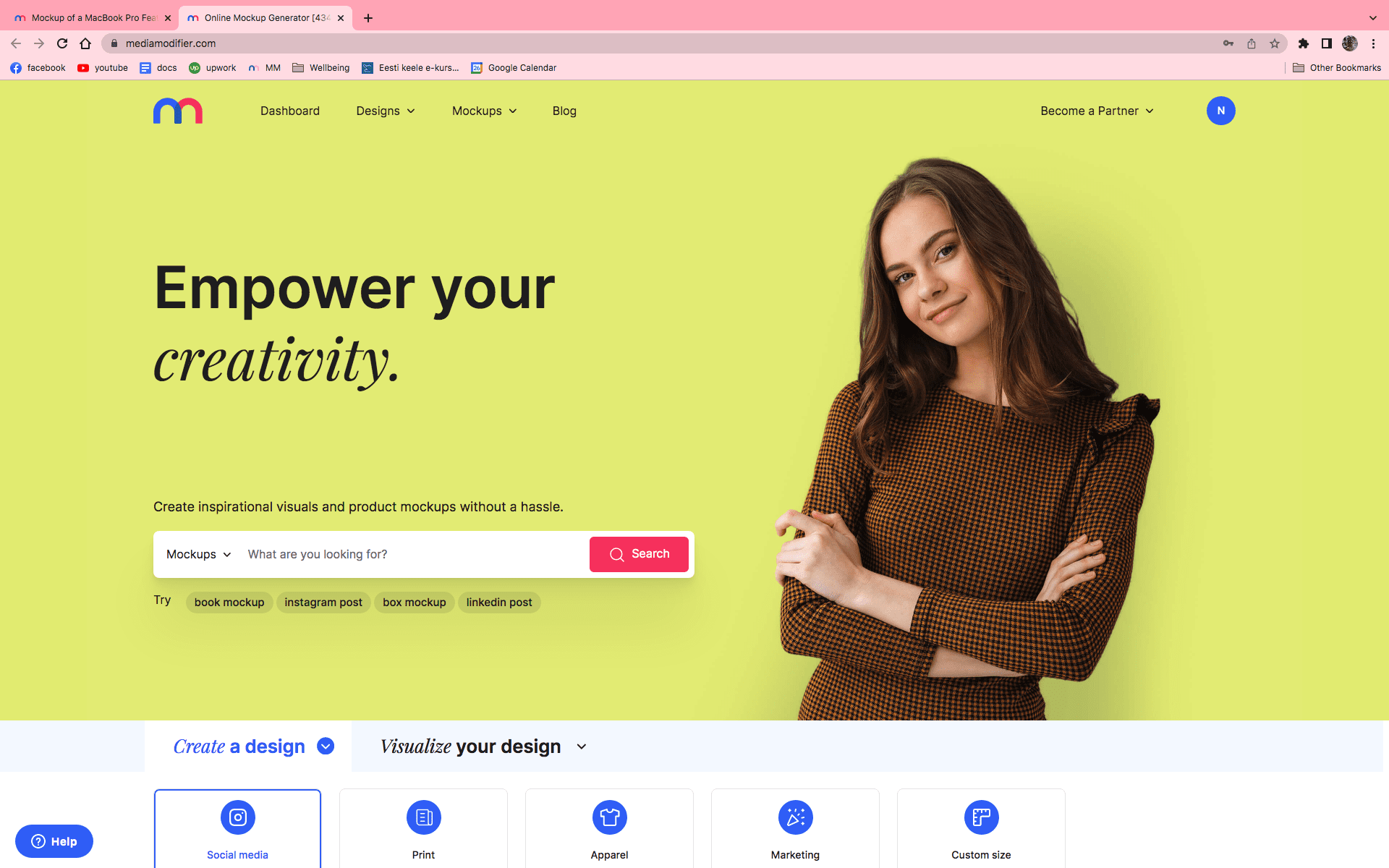The website features a vibrant and colorful design, highlighted by a prominent dark pink navigation bar at the top. This bar includes various browser icons that are somewhat small and difficult to read but contain textual labels. Just below the dark pink bar is a lighter pink one, which houses a gray sub-bar with clickable items, each distinguished by a different color icon such as green, blue, and red.

Beneath this, the site displays a large 'M' logo, split into blue and red halves. Next to the logo, there are options labeled "Dashboard Designs," "Mock-ups," and "Blog," each offering drop-down menus for further navigation. To the right of these options, there is a blue circular button labeled "Become a Partner."

Continuing down the page, a callout section with the text "Empower Your Creativity" features an image of a woman wearing a brown sweater, her arms folded across her chest, her head tilted to one side, and her long brown hair cascading down. Adjacent to this image is a search bar prompting users with the text "What are you looking for?" followed by a red search button labeled "Search."

Below this section, there are suggestions for different clickable options labeled "Try," encouraging users to engage with various features. Additionally, a section titled "Visualize Your Design" offers multiple blue icons for users to explore various design tools and features available on the site.